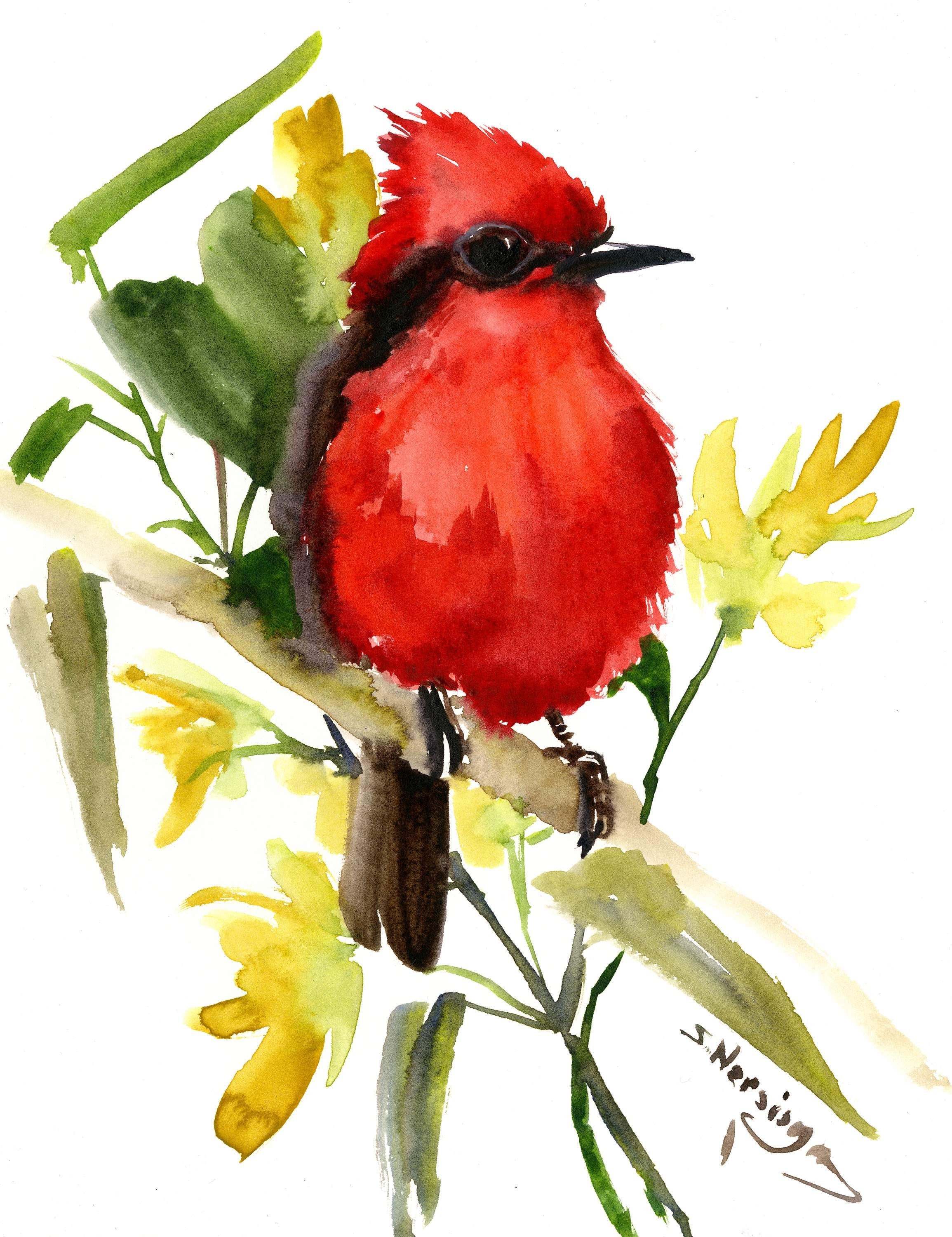This is a detailed watercolor depiction of a small red bird, likely a cardinal, perched on a tannish brown branch amidst vibrant yellow flowers and green leaves. The bird features distinct black eyes, a black beak, and a striking black streak of feathers progressing from its head down to its tail. The use of brushstrokes gives the bird a fluffy appearance, accentuating its rotund form, while the flower petals are rendered with more concrete shapes. The bird is oriented to the viewer's right. Below the branch, the artist has subtly integrated their signature, “S Nursing,” written in black. The image is vertically rectangular with no border, other than the computer screen background.